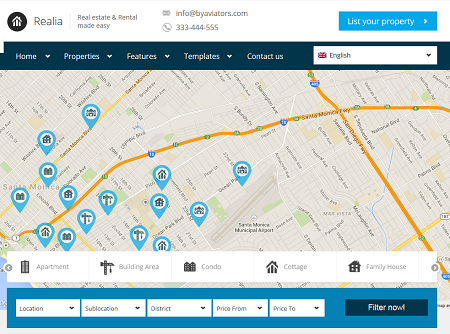**Screenshot Description:**

The screenshot showcases the Renalia website, which focuses on real estate and rental services, with the tagline "Real Estate and Rental Made Easy". The top of the page features an envelope icon labeled "info," along with the website's name, byviatters.com, and a contact number, 333-444-5555, in small print. The navigation bar includes options like "List Your Property," "Home," "Properties," "Features," "Templates," "Contact Us," and a drop-down menu currently set to English.

A prominent map adorned with numerous blue location symbols occupies the center of the screen. Each location symbol includes thumbnail images indicating different property types. Below the map, there's a legend that categorizes these properties with corresponding icons and labels: "Apartment," "Building Area," "Condo," "Cottage," and "Family House."

At the very bottom, a detailed filter section allows users to refine their property search by specifying "Location," "Sublocation," "District," and price ranges ("Price From" and "Price To"). A button labeled "Filter Now!" concludes the section.